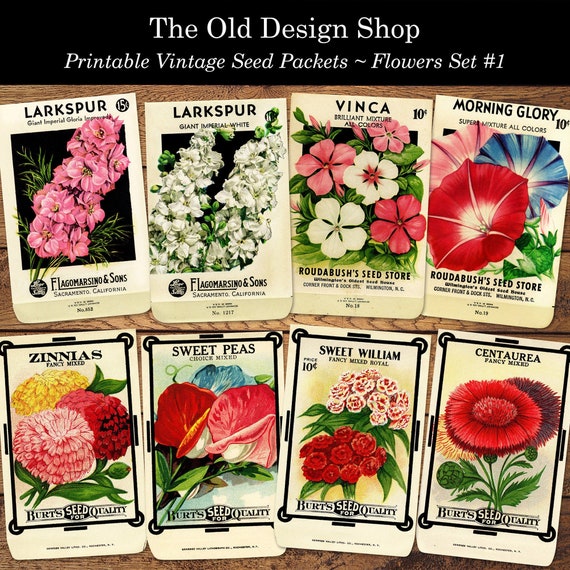The image features a vintage-themed flyer displaying a collection of eight seed packets from "The Old Design Shop," titled "Printable Vintage Seed Packets, Flowers Set Number One." The flyer has a distinct black banner at the top with white text and a rustic wood background. The packets are neatly arranged in two rows of four. Each packet, emblazoned with a detailed illustration of the flower it represents, includes the names and varieties of the seeds, accompanied by additional details at the bottom. The flowers featured are:

1. **Larkspur** from Sacramento, California - One packet with a pink flower and another with a white flower labeled 'Giant Imperial White.'
2. **Vinca** - Showcasing various hues including white, pink, darker pink, and a striking white flower with a pink center.
3. **Morning Glory** - Displaying vivid blooms in red, blue, and pink.
4. **Zinnias** - Featuring colorful blossoms in shades of pink, red, and yellow.
5. **Sweet Peas** - Highlighting floral variations in red, pink, and blue.
6. **Sweet William** - With striking red flowers and a white variant displaying reddish-yellow markings.
7. **Centurea** labeled as 'Fancy Mixed' - Includes diverse flowers in yellowy, red, and dark purple-burgundy tones.

These seed packets are attributed to iconic seed suppliers like Burt’s Seed for Quality, Lago Moricino and Sons, and Rhoda Bush's Seed Store, all set against a white backdrop emphasizing their vintage appeal.